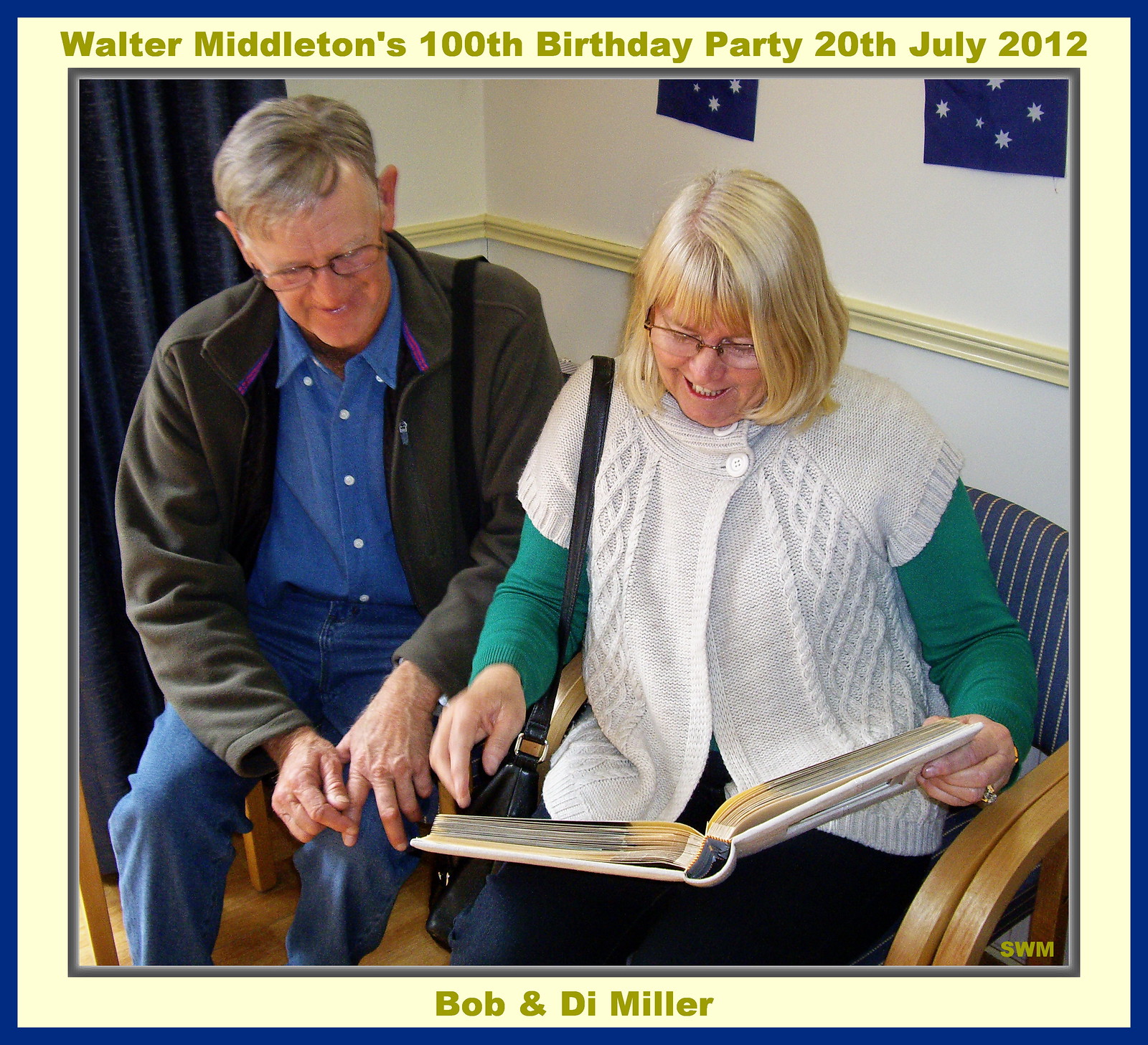This photograph showcases an elderly couple seated side-by-side, engrossed in a photo album held by the woman. The picture is framed by a virtual border, with inscriptions above and below noting, "Walter Middleton's 100th birthday party 20th July 2012" and "Bob and Dee Miller." The couple appears to be in their 60s, wearing glasses and seated in front of a white wall with yellow molding. The woman, with shoulder-length blonde hair, wears a long-sleeve green shirt layered with a white short-sleeve cover and blue jeans, complemented by a black purse on her right shoulder. She sits on a blue chair with yellow stripes and wooden armrests. The man beside her sports grayish hair, a blue button-down shirt, blue jeans, and a brown jacket. Behind them is a blue curtain, adding a touch of color to the setting. The photograph captures a serene, intimate moment, highlighting the warmth and connection between the two.